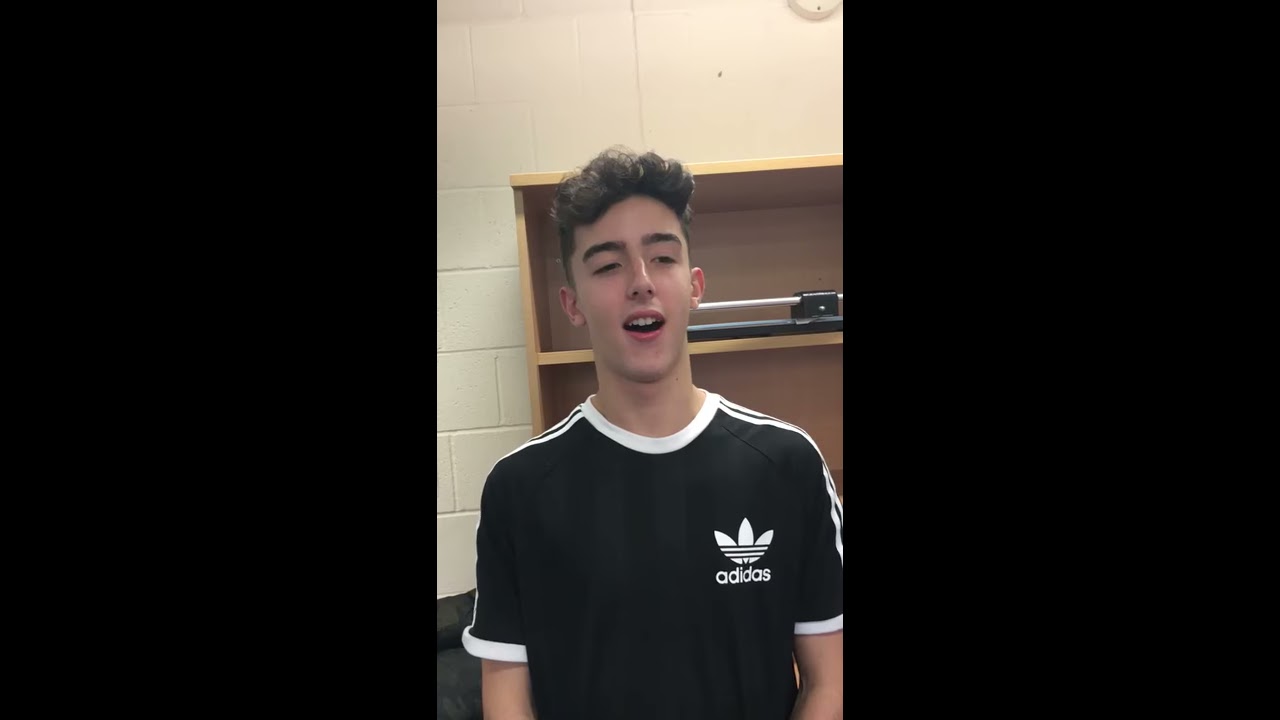The image features a young man, likely a teenager or in his early twenties, standing in front of a beige, cinder block wall with a white-brick pattern. He is wearing a black short-sleeved t-shirt with white Adidas branding on the left chest and signature white stripes on the shoulders and neck. The young man has brown hair and is looking directly at the camera. Behind him, there is a brown cabinet with three shelves; the top shelf contains an indistinguishable item, while the second shelf has something on it and the bottom shelf is empty. In the upper right corner of the image, only the bottom half of a wall-mounted clock is visible. Additionally, a smoke alarm is present on the wall above the man's left shoulder.